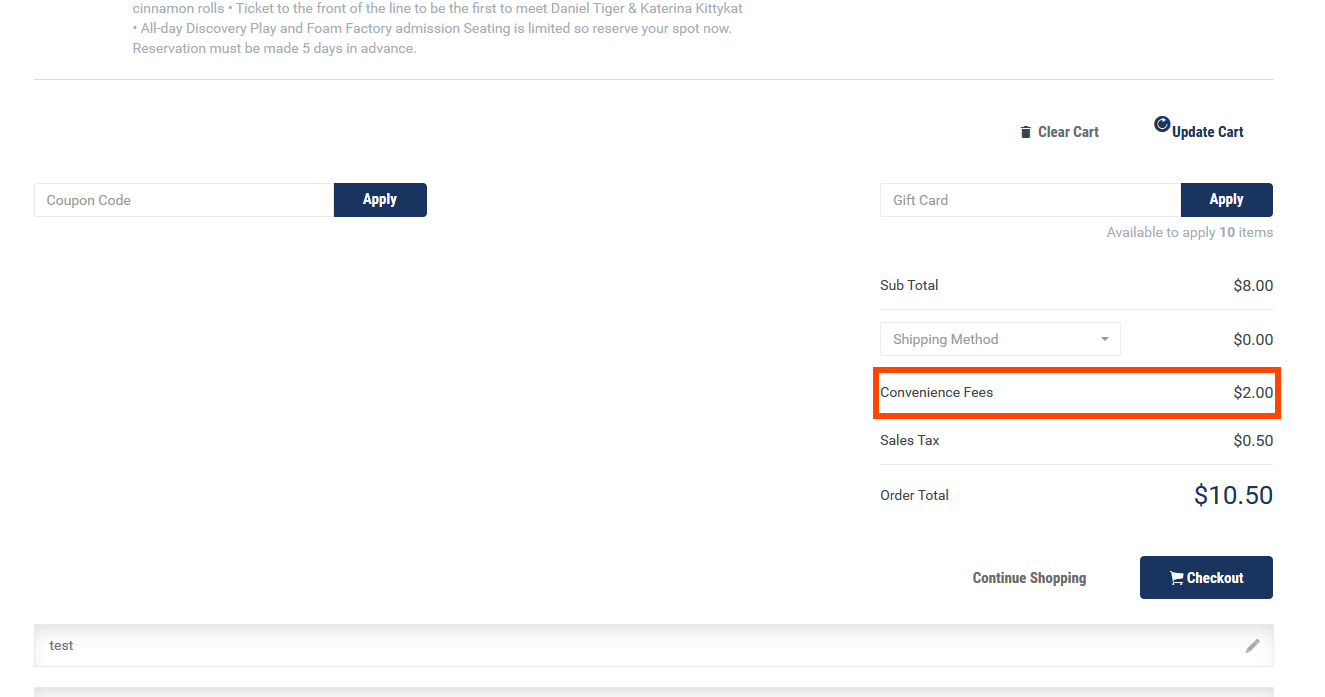This is a detailed screenshot of a website's shopping cart checkout page. At the very top of the screen, in small print, it lists:

- "Cinnamon Rolls"
- "Ticket to the front of the line to be the first to meet Daniel Tiger and Katerina Kitty Cat"
- "All-day Discovery Play and Foam Factory admission"
- A note that "Seating is limited so reserve your spot now. Reservations must be made five days in advance."

Below this text, there is a coupon code field accompanied by an "Apply" button to its right. On the right side of this window, users can find an "Update Cart" button and a "Clear Cart" button. There's also a section for entering a gift card code, followed by another "Apply" button.

The cost breakdown is displayed as follows:

- Subtotal: $8.00
- Convenience Fee: $2.00
- Sales Tax: $0.50
- Order Total: $10.50

At the bottom right corner of the screen, there are "Continue Shopping" and "Checkout" buttons.